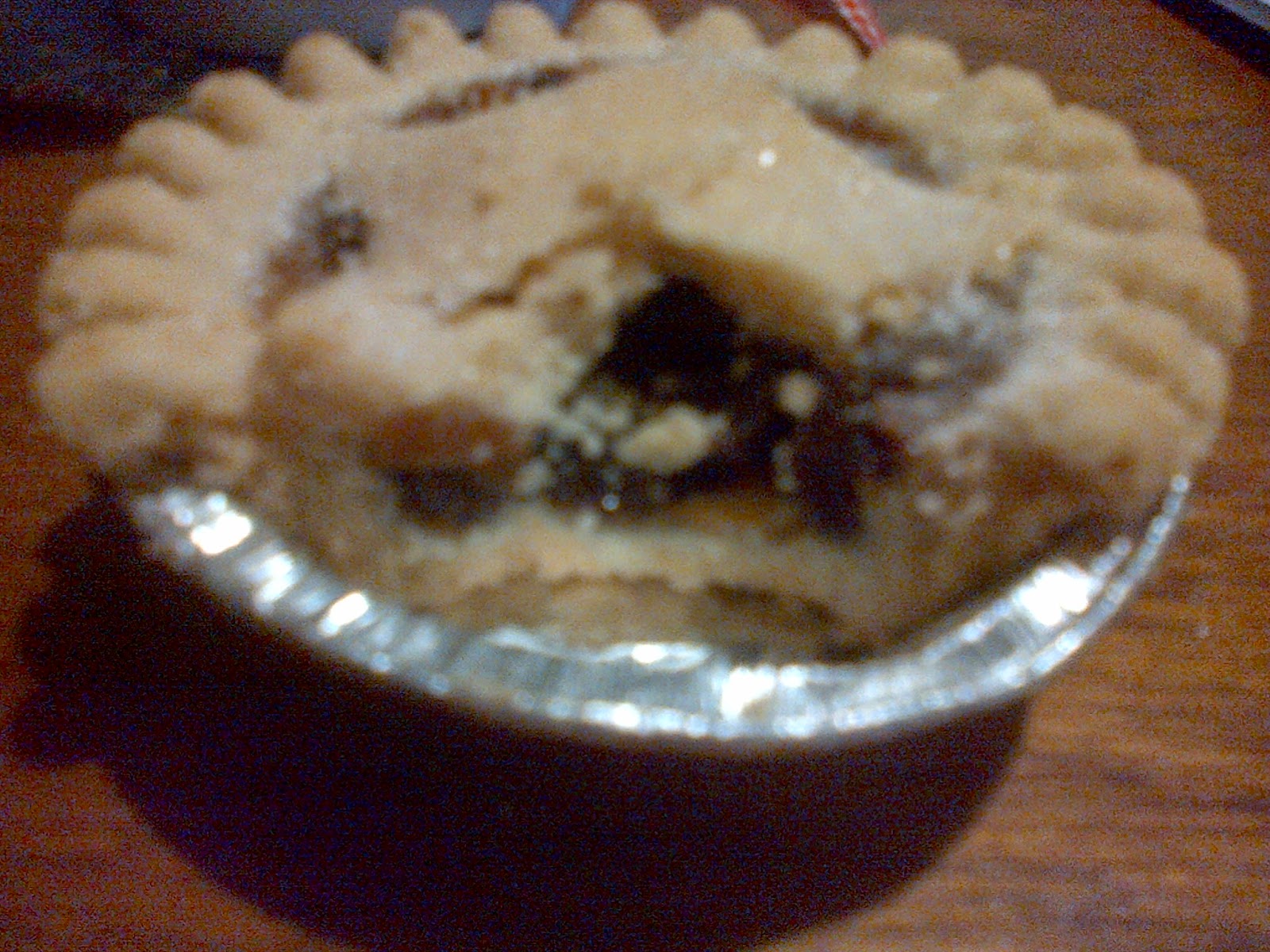The image features a small, single-serving pie placed in a lightweight silver metal pie tin, sitting on an aged, deep brown wooden table. The pie has a golden brown, flaky crust with fluted ridges around the edges and a slightly irregular opening at the top, revealing a dark filling that resembles mincemeat or perhaps a dark caramel or amber filling, although it’s difficult to determine precisely. A bite has been taken out of the pie, showing a rough, uneven edge. The light source appears to come from directly above, casting a shadow at the lower edge of the pie tin. The photograph is slightly blurry, and there are additional, indistinct objects placed on the table in the background.